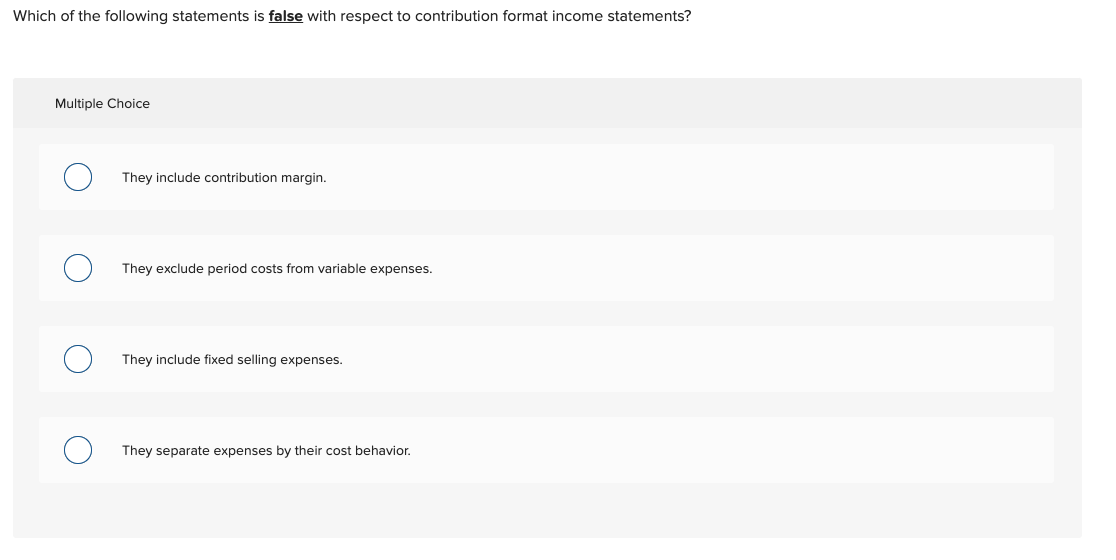The image depicts a section of a web page designed as a multiple-choice question. At the top of the page, a question is displayed in standard text, which reads, "Which of the following statements is false?" Notably, the word "false" is bolded for emphasis. Below the question is a rectangular gray box, which serves as the container for the multiple-choice options.

Within this gray box, the term "Multiple Choice" is positioned at the top left. There are four horizontally-aligned multiple-choice options, each with an unselected circular button on their left, outlined in blue with a white interior. 

The multiple-choice statements are as follows:
1. "They include contribution margin."
2. "They exclude period costs from variable expenses."
3. "They include fixed selling expenses."
4. "They separate expenses by their cost behavior."

Each of these statements is situated in a white area within the gray box to maintain readability. Users can select an answer by clicking the corresponding circle next to each statement. The overall background of the web page is white.